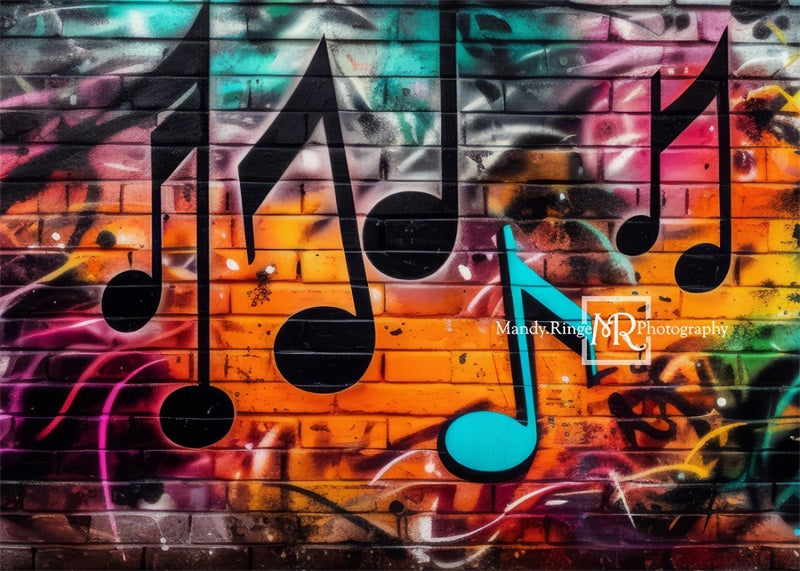This horizontally oriented image showcases a digitally-generated or artistically drawn depiction of a brick wall meticulously painted to appear almost factory-produced, presenting no gaps in its vibrant and detailed paint job. The primary background consists of brick patterns seamlessly blended with shades of yellow, orange, pink, green, blue, and purple, forming an abstract and artistic design. Overlaying this colorful graffiti are a series of five musical notes rendered mostly in black, with a standout turquoise note, accented with black shading, positioned towards the bottom right middle of the image. At the center, a watermark reads "mandy.ringe photography," accompanied by a logo featuring the initials "MR," encapsulated within a square.